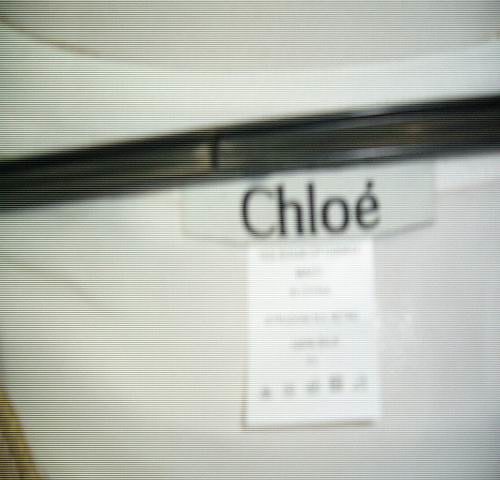The image shows a highly zoomed-in view of the back side of a shirt or dress collar, highlighting two tags against a slightly blurred background. The shirt itself is white with faint horizontal lines across the fabric, giving the impression that the photo was taken from a screen. The top tag is a horizontal rectangle with a white background that prominently reads "Chloe" in black letters. Below it, a vertical white tag displays washing instructions and material information, although their exact details are unreadable due to blurriness. The tags are attached near a thin leather strip that lines the top of the collar area. At the very top of the image, a black plastic band—possibly a part of a hanger—is visible, adding an interesting element to the composition. Additionally, a bit of tan material appears in the bottom right corner, with a white backdrop resembling a table visible at the top.